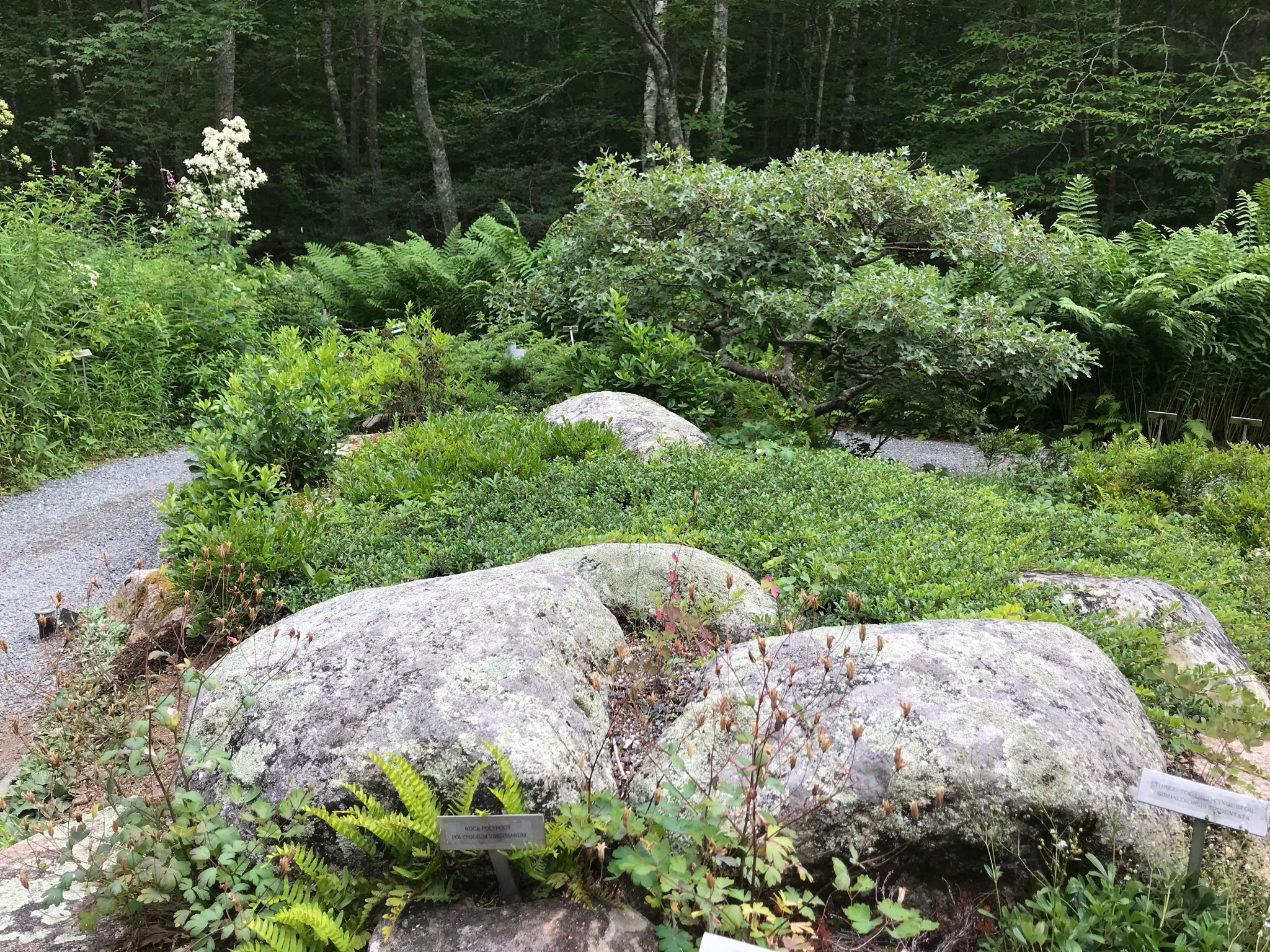This photograph captures a lush, garden-like area, possibly part of a park or arboretum, situated in front of a dense forest. Central to the image are two large, rounded gray rocks positioned at the bottom left and right of the frame, with a variety of green vegetation, including identifiable ferns and other hardy plants, densely filling the space between them. Small white signs, likely indicating plant species, are placed in front of these rocks and another sign is faintly visible poking up in the middle of the scene. To the left, a gravel pathway curves up and to the right, passing beyond the rocks and extending off the image's right-hand side. This path is bordered by additional greenery, flowers, shrubs, and what appears to be a modern-looking tree reminiscent of a bonsai. Purple flowers are noticeable in the foreground, contrasting with the dominant greenery. The background features a dense row of tall trees with gray trunks, enhancing the natural, serene ambiance of this meticulously landscaped area.